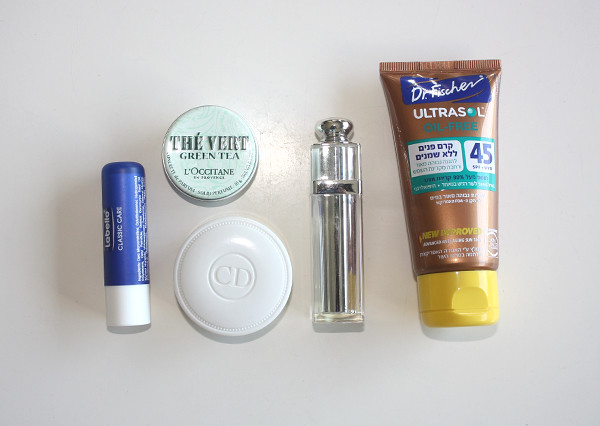This photo captures an elegant arrangement of five skincare and face products displayed on a pristine white table, illuminated by both natural and artificial light. The artificial light source, positioned directly above the table, casts a small shiny spot creating an eye-catching highlight on the surface. Complementing this, natural light filters in from a nearby window, enriching the scene with a soft, diffused glow.

On the far left, there's a chapstick with a distinctive white base and a blue cap. The chapstick is open, revealing its clear balm. The label reads "Labello Classic Care" and is accompanied by a list of ingredients.

Next to the chapstick, two round containers are aligned vertically. The top container, labeled "L'Occitane Thé Vert Green Tea," features an image of green tea leaves on its light green lid, suggesting it might be a lip balm. Below this, another round container displays the letters "CD," hinting at a high-end product, possibly from the Dior brand, though its exact purpose remains ambiguous.

The fourth item in the lineup is a sleek, silver tube, likely a sample-sized perfume. It is elegantly designed with a smooth cylindrical body and topped with a small, round cap.

Finally, the last product is a bottle of "Dr. Fisher Ultra Sol Oil-Free" sunscreen, as indicated by the partially visible "SPF 45" label. Despite some glare obscuring part of the text, it's clear that the bottle combines both English and Asian characters. The bottle is brown with a contrasting yellow cap, rounding out this curated selection of skincare essentials.